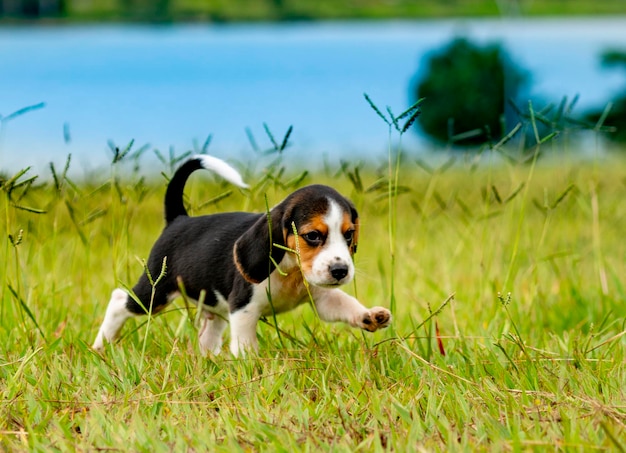In this horizontally aligned rectangular picture, a beagle puppy is captured in mid-run through a field, giving a lively and determined impression. The small pup's main body is predominantly black with white on his underside and front paws, as well as around his ankles and the tip of his tail. His head is a mixture of colors: black covers the top and long, floppy ears, while light brown surrounds his eyes and edges the ears. A white streak begins from his forehead, extending down the sides of his mouth and snout, emphasizing his expressive eyes and black nose. 

The puppy's left front paw is raised as he runs towards the right, his tail arched in an interesting shape. The field consists mostly of short green grass speckled with taller blades, with patches of brown soil visible here and there. In the background, partially blurred, is a body of water with hints of greenery above it, possibly indicating a pond. Overall, the image showcases a cheerful and energetic puppy enjoying a playful run through a grassy field, perhaps captured by his owners.